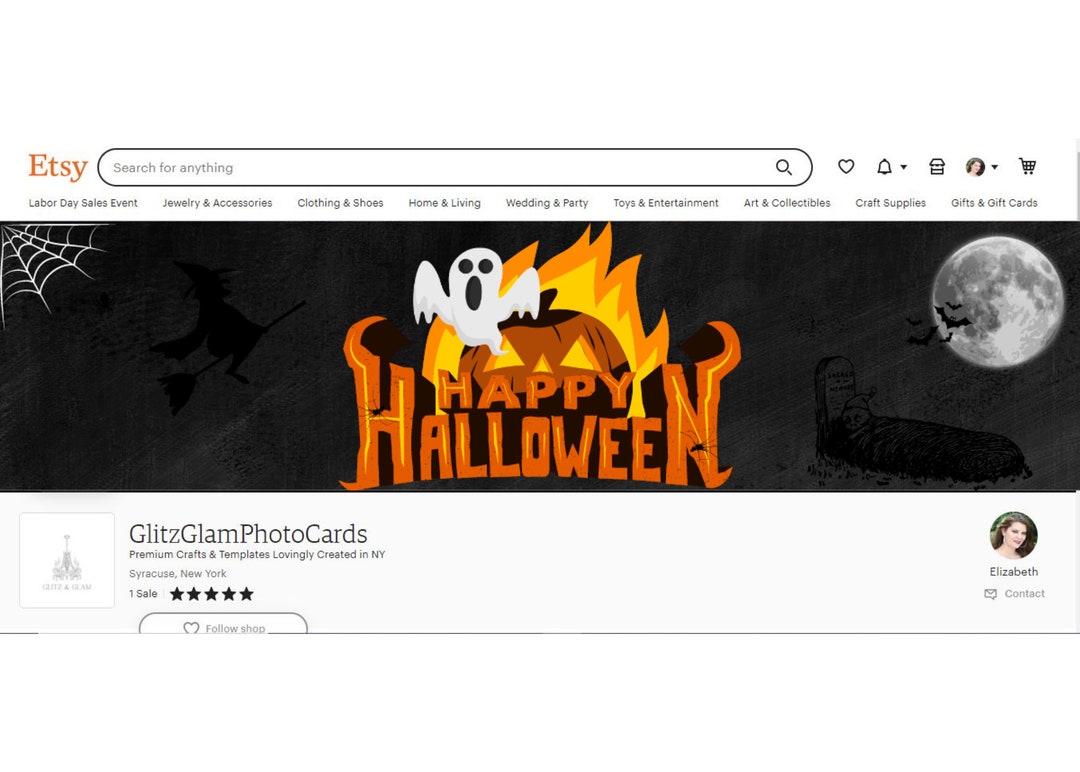A detailed caption for the described Etsy webpage could be:

---

The Etsy homepage showcases a user-friendly interface with a prominent search bar at the top center, inviting visitors to "Search for anything." To the right of the search bar, you'll find a heart icon for favorites, a notifications bell, and an account profile picture, which in this case belongs to a user named Elizabeth, located towards the lower section of the page.

A festive banner stretches across the width of the page, celebrating Halloween with the message "Happy Halloween." This message is creatively styled with horns on the "H" and upward-curving "N"s, adding a spooky flair. The banner is decorated with a cartoon ghost, a flaming pumpkin, and a spider web in the upper left-hand corner. Interestingly, a realistic photograph of the moon, featuring bats flying in front of it, contrasts with the otherwise cartoonish theme.

Beneath the banner, there's a promotional section for "Glitz Glam Photo Cards," highlighting premium crafts and templates lovingly created in New York. Accompanying this text is an image of one of the photo cards, alongside the mention that it is from Syracuse, New York, and has received a 5-star rating from customers. Additionally, there's a button allowing users to follow the card creator.

To the right, the page indicates that the user Elizabeth is signed in, with her profile picture displayed. There is also an option to contact Etsy, humorously mislabeled here as "Etsy Betsy," to inquire about selling your own items on the platform.